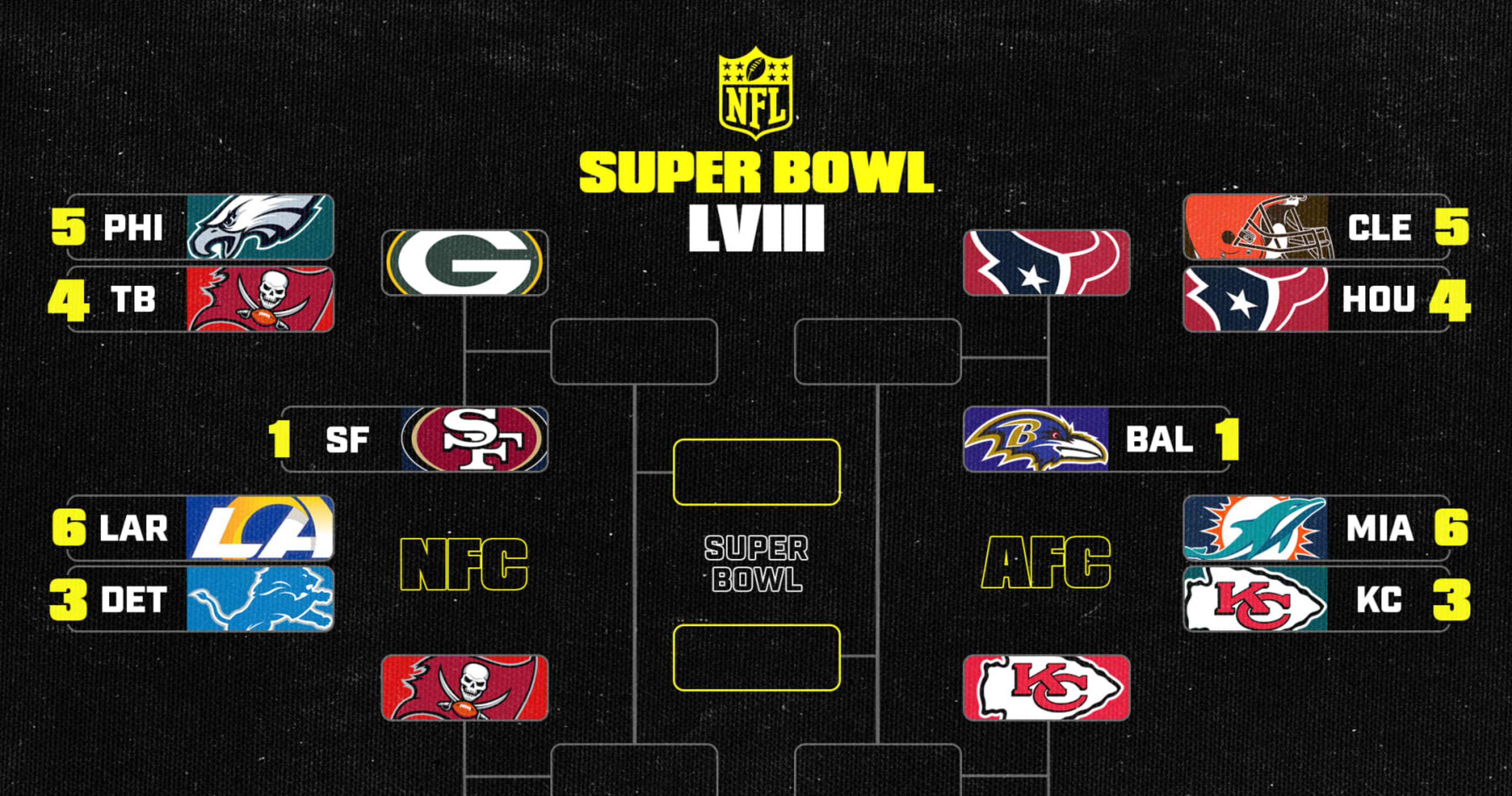This image is a detailed graphic of the NFL Super Bowl LVIII bracket. At the top center, the NFL logo is prominently displayed in yellow, followed by "Super Bowl" in bold yellow letters underneath. Beneath that, the Roman numerals LVIII are in white. The background of the graphic is black, resembling a night sky with tiny stars scattered throughout. The bracket itself is divided into two sides, each labeled for the respective conferences: NFC on the left and AFC on the right.

On the NFC side, the bracket lists team logos and names including Philadelphia (PHI), Tampa Bay (TB), Green Bay (GB), San Francisco (SF), Los Angeles (LA), and Detroit (DET). Similarly, the AFC side shows team logos and names such as Texas (HOU), Cleveland (CLE), Baltimore (BAL), Miami (MIA), and Kansas City (KC). The arrangement includes the first round, second round, and blank boxes for subsequent rounds leading up to the Super Bowl.

In the center of the poster, there are two yellow boxes positioned to represent the final Super Bowl matchup, with the word "Super Bowl" written between them, indicating where the concluding teams will be showcased. This intricate layout allows one to visualize and predict the path teams must take to reach the Super Bowl.